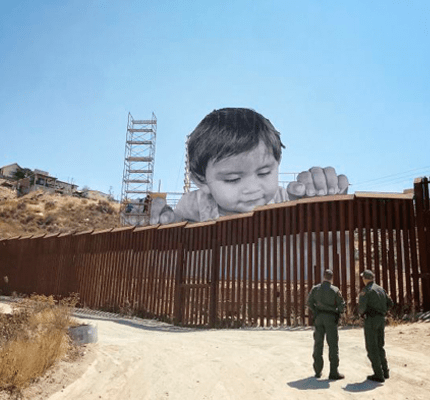The image captures a striking scene at the border wall between America and Mexico. The brown wall, characterized by its vertical bars, stretches horizontally across the entire frame. Standing on a dusty dirt road are two men in dark green full-body suits and hats, likely border patrol agents, gazing up at a large black-and-white image of a child. The child's massive hands rest atop the wall, and the child peers down at the two men, suggesting a powerful political art installation. To the left, scaffolding is visible near some dried vegetation and a metal tower, and in the background, tan hills dotted with buildings rise under a clear, bright blue sky. The image evokes a sense of starkness and contemplation, highlighting the separation and the human element within a landscape defined by boundaries.